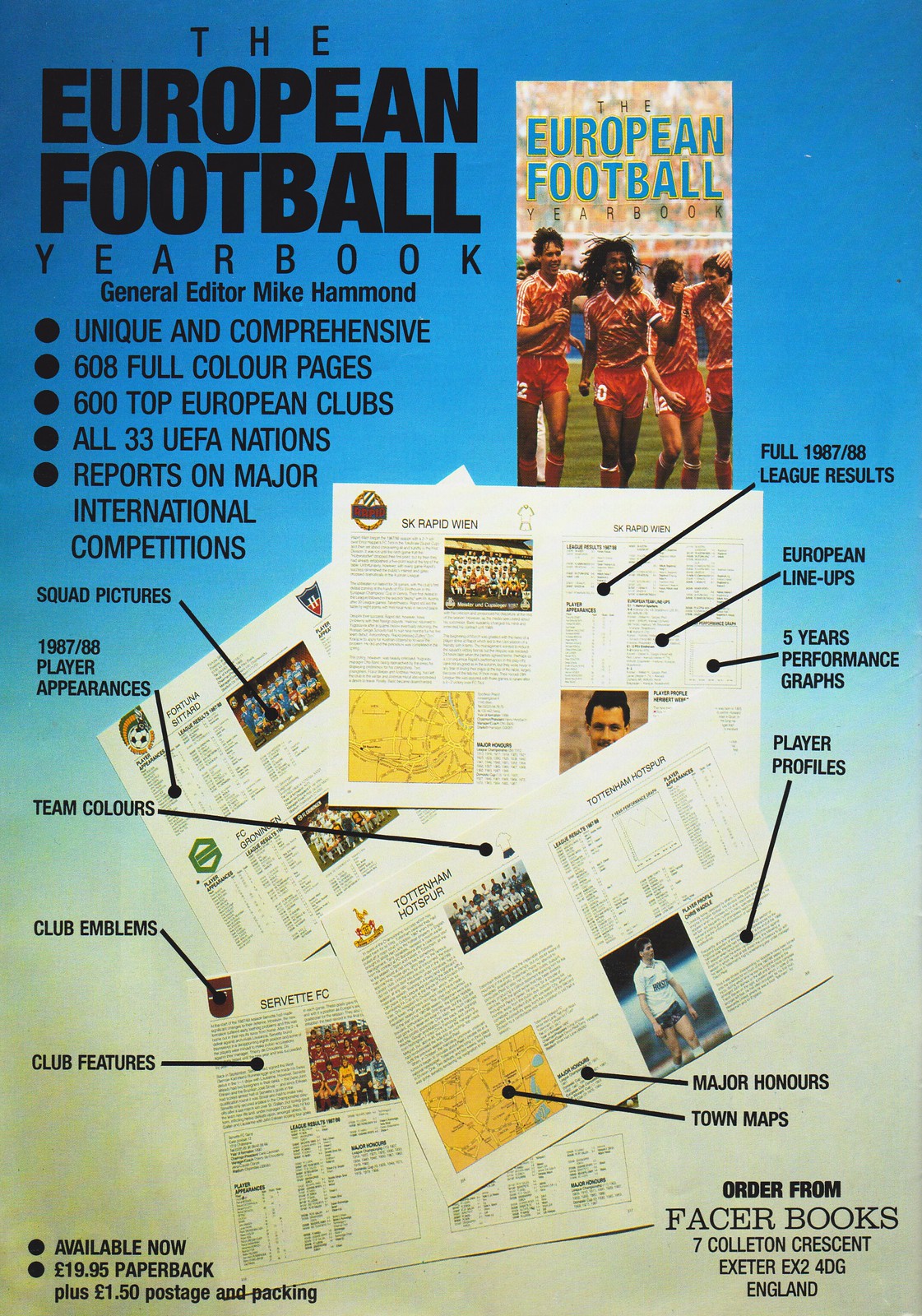This is a color image of the cover of the "European Football Yearbook." The background features a blue gradient that transitions to a greenish-yellow hue at the bottom. In the upper left-hand corner, bold black text declares "The European Football Yearbook," followed by the name of the General Editor, Mike Hammond, and several bullet points highlighting the book's features: "Unique and comprehensive," "608 full-color pages," "600 top European clubs," "All 33 UEFA nations," and reports on major international competitions. To the right of this text is an image of football players in red uniforms, appearing to cheer together on a field, with people in the background. Below this, the cover showcases an assortment of the yearbook's pages, highlighting sections such as squad pictures, player appearances for 1987-88, team colors, club emblems, club features, full league results, European lineups, five-year performance graphs, player profiles, major honors, and town maps. In the lower section, a note reads "Available now for £19.95 plus £1.50 postage and packing." The business details are located at the bottom right corner: "Fazer Books, 7 Colleton Crescent, Exeter, EX2 4DG, England."